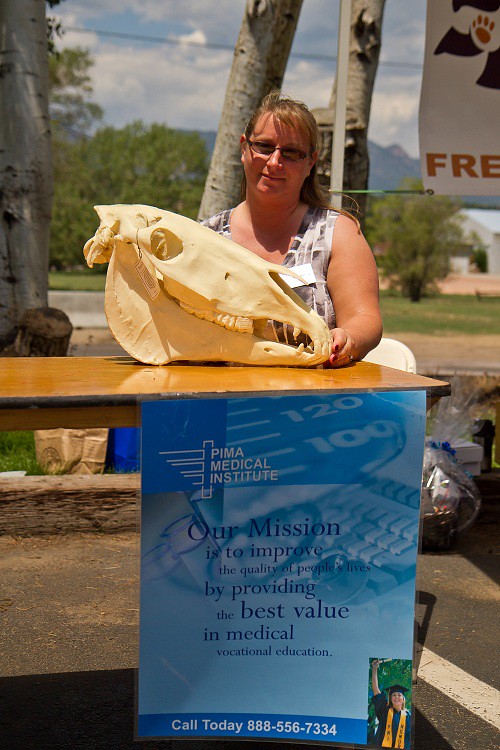In the photograph, a woman with blondish-brown hair, pulled back and wearing sunglasses, is posing with a large animal skull, likely a cow or bull skull. The skull, a light yellow color, is placed on a folding table adorned with a prominently displayed blue poster. The poster, with white and blue text, reads, “Pima Medical Institute. Our mission is to improve the quality of people's lives by providing the best value in medical vocational education. Call today, 888-556-7334.” The woman is dressed in a sleeveless top, suggesting a warm outdoor environment, accentuated by the visible pine trees and open sky in the background. A small image of a jubilant graduate with a gold collar, mortar board, and raised hand can be seen on the lower right-hand corner of the poster, adding to the festive and informative ambiance of the scene. Some paper and plastic bags are also visible around the table, hinting at a casual, possibly fair-like setting.